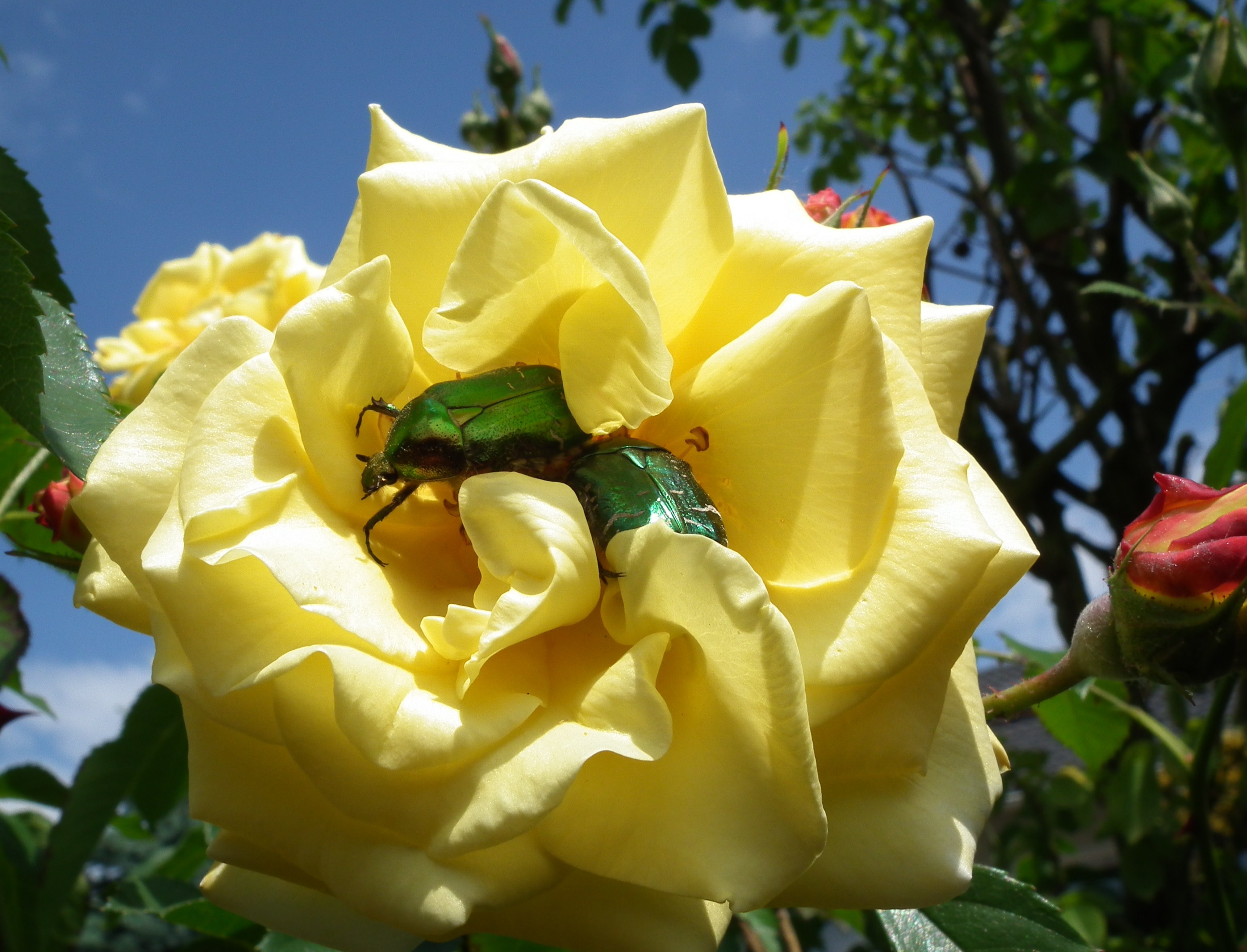This is a detailed, close-up photograph of a stunning yellow rose set against a backdrop of a clear blue sky with scattered white clouds. The vibrant yellow petals dominate the center of the frame, displaying layers upon layers of bright colors. Nestled within the heart of this rose, two large green beetles with shiny, metallic-like shells are visible. One beetle's head and front legs are prominently displayed, while the body of the other beetle can be seen beside it, creating a striking and slightly unsettling focal point. Surrounding the primary yellow rose, additional flowers, including red and orange buds, are interspersed. On the upper right, a tree with green leaves and branches adds to the vibrant, natural setting.